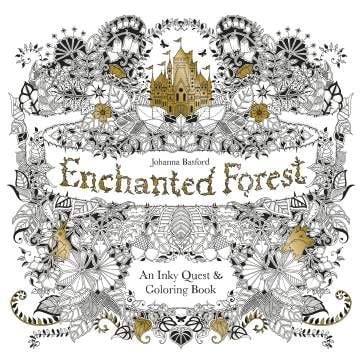This image is the front cover of a coloring book titled "Enchanted Forest" by Johanna Basford. The cover features an intricate, hand-drawn pen and ink design with a whimsical, nature-inspired theme. Central to the cover is a white rectangular background where the title "Enchanted Forest" appears in a gold-greenish, vine-like font, contributing to the overall earthy and enchanting vibe. Above the title, the author's name is presented in a simple, elegant font. The design includes a gold castle at the top center, flanked by golden leaves on the right and two golden flowers underneath. At the bottom, the words "An Inky Quest and Coloring Book" are highlighted, with additional gold leaves and flourishes enhancing the black and white floral and foliage motifs. The cover, with its detailed leaves, flowers, acorns, and tiny elements, emphasizes the complex and sophisticated patterns found inside, suggesting this coloring book is aimed at adults.